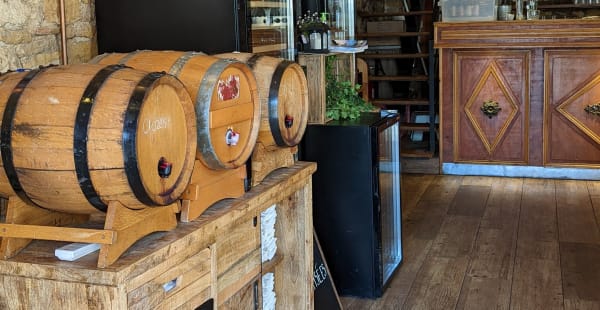The photograph depicts an interior space, possibly a living room or a store, featuring a mix of rustic and contemporary decor. To the left, an old wooden dresser with a few drawers and shelves is visible. The shelves contain white cloths, and atop the dresser, three small to medium-sized brown barrels with spouts are arranged diagonally on stands, each secured with steel rings. Behind the barrels, a black mini fridge with a glass front stands, adorned with a green plant. The wall behind these items is constructed of tan stone, adding to the rustic charm.

The floor consists of large planks of medium to dark brown hardwood, evoking an older, more traditional style. In the upper right-hand corner, a wooden bar counter is visible, decorated with triangular and diamond carvings along its side. Adjacent to the bar, there are wooden shelves, albeit sparsely filled. The overall setting combines a cozy, old-world ambiance with functional modern elements.